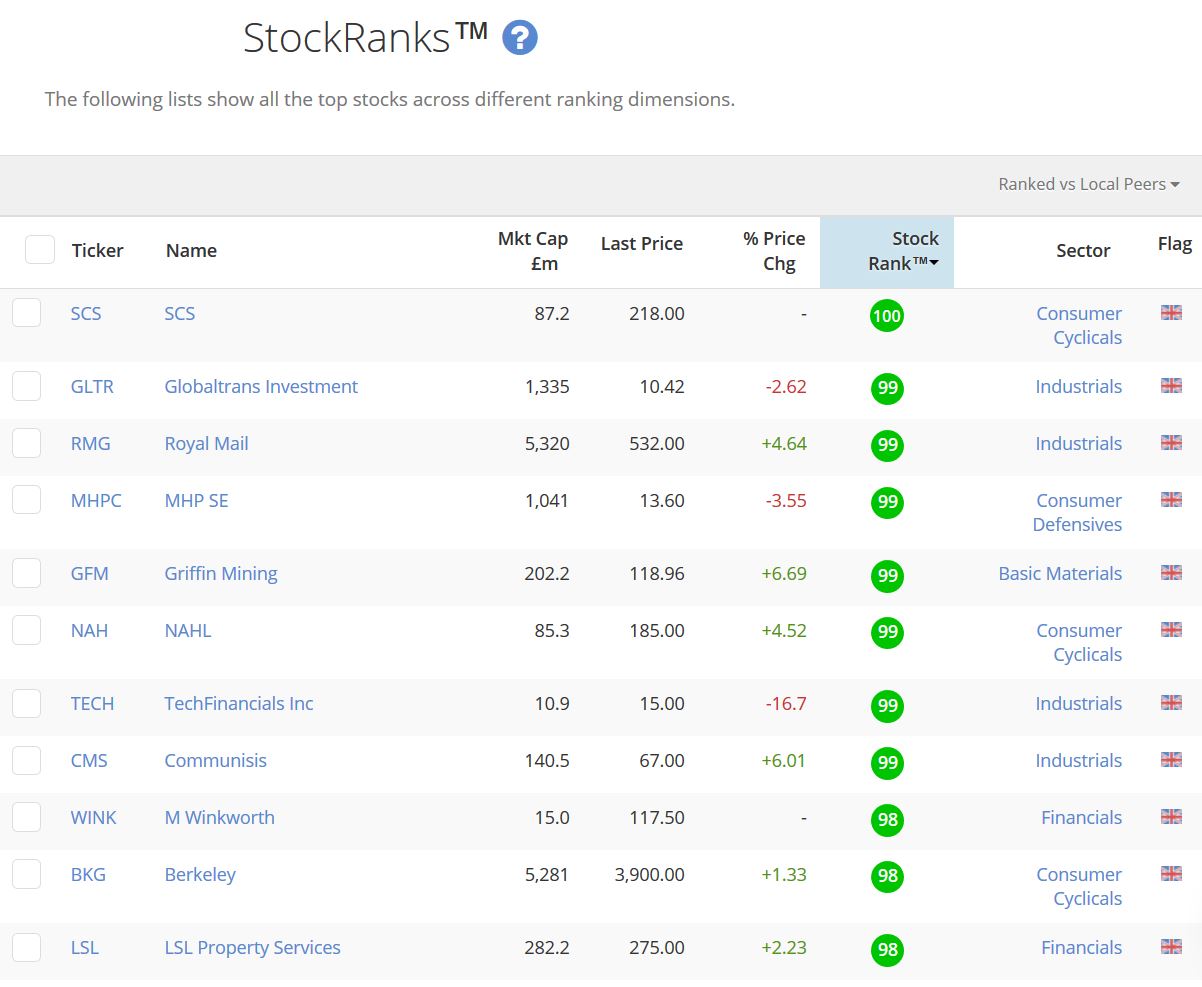This image showcases a comprehensive list of top-ranking stocks evaluated across various dimensions. The upper section highlights a ranking comparison versus local peers, with rows of stocks denoted by tickers, accompanied by attributes such as name, market cap, last traded price, price change percentage, and overall stock rank. Each stock entry also includes a sector flag, predominantly British, signifying the origin or main market of the stock. The list is numerically ordered from 1 to 11, with unchecked boxes next to each stock ticker indicating their selection status. This meticulous layout provides an in-depth comparison and facilitates easy identification of high-performing stocks in different sectors.